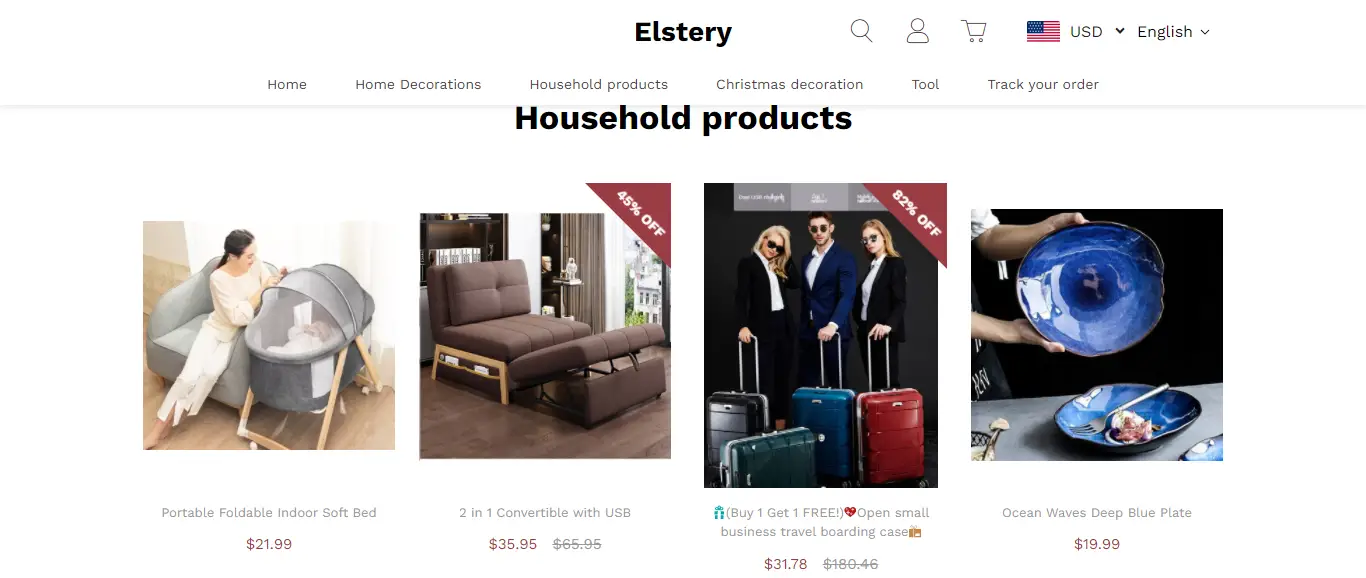On the Elstery web page, the title "ELSTERY" is displayed prominently at the top center in bold black ink. Adjacent to it are icons for search, account access (depicted as a small head and torso), shopping cart, U.S. flag, currency dropdown (USD), and a language dropdown (English). The navigation menu below includes options for Home, Home Decorations, Household Products, Christmas Decorations, Tools, and Track Your Order.

Currently within the "Household Products" section, several items are showcased: 

1. A portable, foldable indoor soft bed priced at $21.99, illustrated with an image of a lady standing next to a bassinet.
2. A 2-in-1 convertible recliner with USB functionality, available for $35.95.
3. An advertisement featuring a man flanked by two women, all dressed in business attire, with four suitcases (three rollable) in front of them, promoting a buy one, get one free deal on small business travel boarding cases for $31.78.
4. A striking "Ocean Waves Deep Blue Plate," which resembles a shallow bowl with a blue swirled marble design, listed at $19.99.